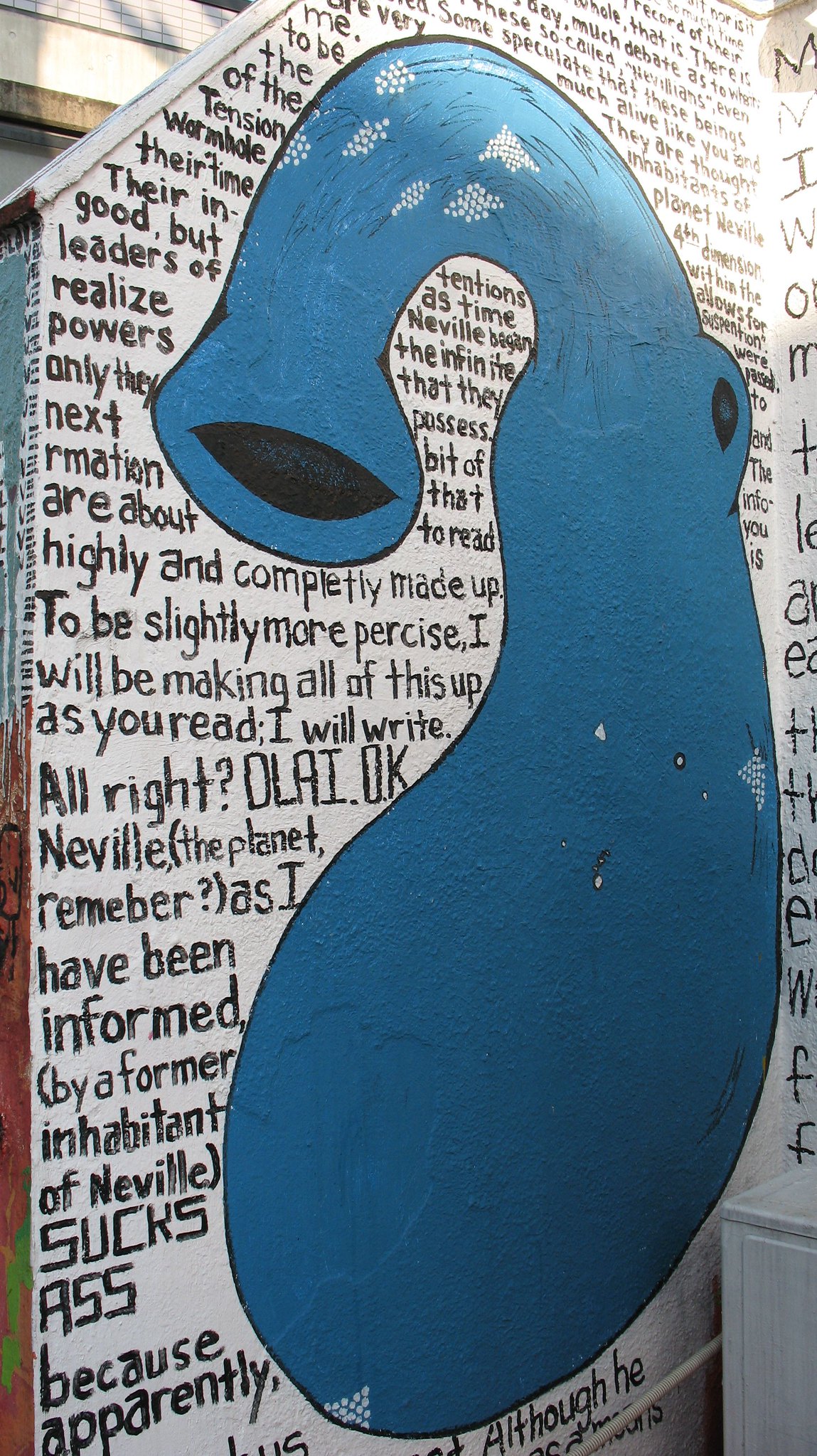The image features an exterior wall resembling a staircase, with a backdrop painted in white. The wall isn’t perfectly square; its top left section slopes down instead of forming a right angle. Dominating the center of this wall is a striking piece of mural art depicting a large, deep bright blue creature. This creature bears a resemblance to a blend of an elephant and an octopus, characterized by a long trunk-like nose extending to the left, adorned with white dotted patterns. The creature has a black eye situated on the right side of its body. Surrounding the blue creature, every portion of the white wall is covered in black text, forming a dense tapestry of words and sentences that give the impression of a fragmented story or chaotic narrative. Some sections of the text read: "D-Lad, okay. Neville, the Planetary Member, as I have been informed by a former inhabitant of Neville, sucks ass because apparently...". This extensive text seems scattered and haphazard, with numerous spelling errors adding to the chaotic feel of the scene.